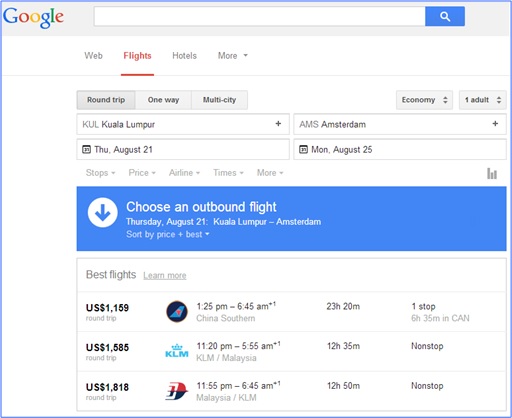The image is a detailed screenshot of a Google Flights search page. At the top left corner, the familiar Google logo is prominently displayed, followed by a large, empty search bar stretching across the page. Below the search bar are four navigation tabs labeled "Web," "Flights," "Hotels," and "More," with "Flights" highlighted in red, indicating the active tab.

Proceeding further down, three tabs labeled "Round-trip," "One-way," and "Multi-city" are visible, with "Round-trip" selected by default. Next to these tabs, the search options specify "Economy" class and "1 adult." Directly beneath this, there are two text entry boxes: the first one labeled "KUL," representing Kuala Lumpur, and the second one labeled "AMS," representing Amsterdam.

Further down, two boxes featuring calendar icons show selected travel dates: Thursday, August 21 for the departure and Monday, August 25 for the return. Below these dates, a set of filter tabs labeled "Stops," "Price," "Airline," "Times," and "More" provide options to refine the search results.

Prominently displayed beneath the filters is a blue box marked with a downward-pointing arrow, prompting users to "Choose an outbound flight." The prompt repeats the selected departure details: Thursday, August 21, from Kuala Lumpur to Amsterdam. There is an option to "Sort by price or best."

The search results are presented in a table format below, listing three flight options. Each option is divided into columns displaying the price in USD, the airline's icon, departure and arrival times, the airline's name, the total flight duration, and whether the flight has any stops or is non-stop.